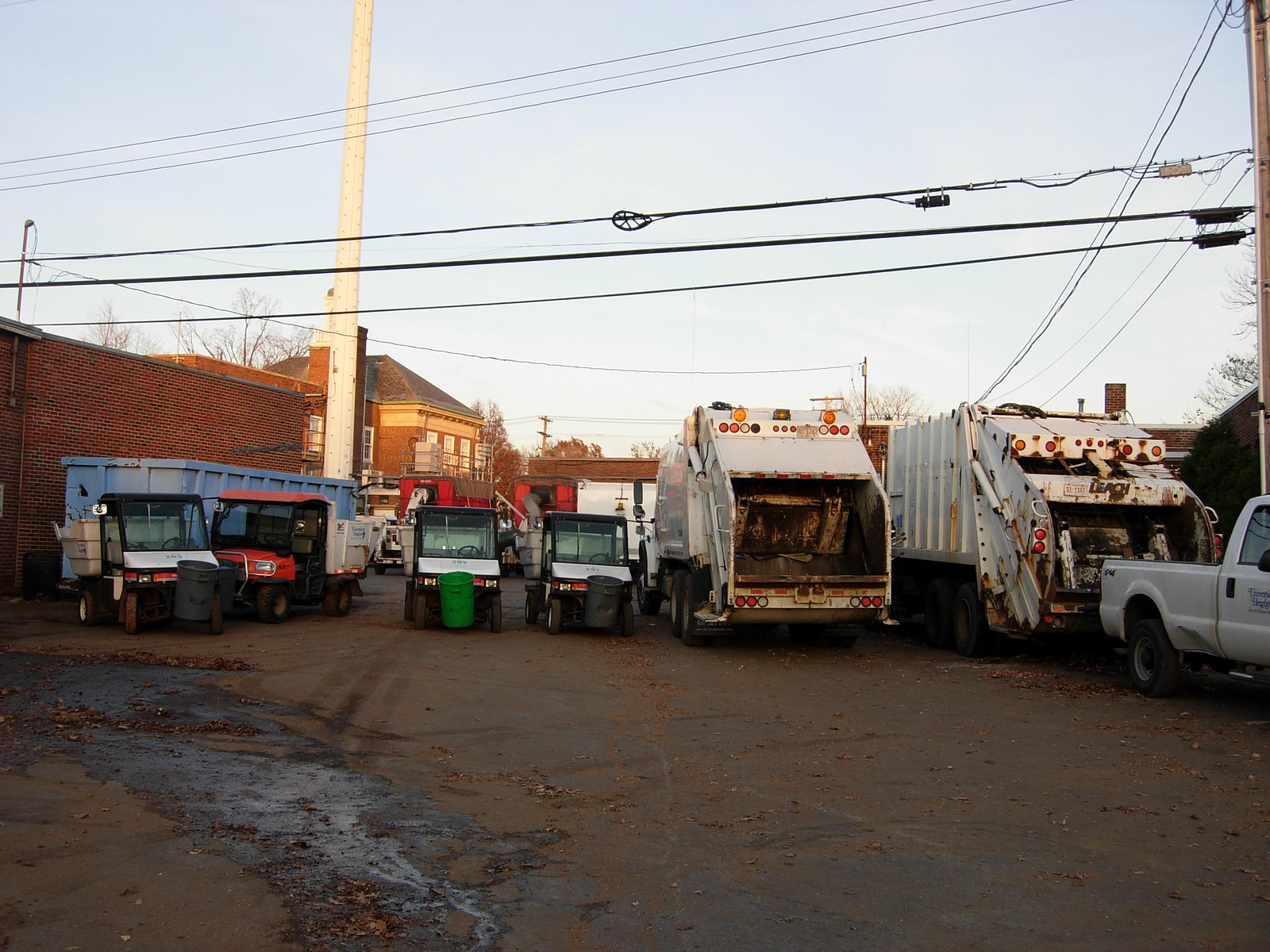The photograph appears to be taken outdoors in a lot or yard used by a garbage collection company. The image captures a mix of vehicles and equipment arranged on what seems to be a concrete or dusty surface with scattered brownish leaves and wet streaks suggesting recent rain or water flow. Dominating the center are two white garbage trucks seen from the rear, with another white utility vehicle parked end-to-end with one of them on the far right. To the left of these trucks are four smaller vehicles resembling golf buggies but designed for trash collection, each equipped with a front-mounted trash can and a tray for rubbish. Further to the left, behind these smaller vehicles, is a large light blue dumpster or skip. In the background to the left and right, buildings can be seen under a pale blue sky with hints of early morning or late afternoon light, while power lines crisscross the sky horizontally, connecting to poles that extend up into the frame. The setting is likely a parking or staging area for trash collection vehicles, providing a utilitarian and slightly cluttered urban landscape.